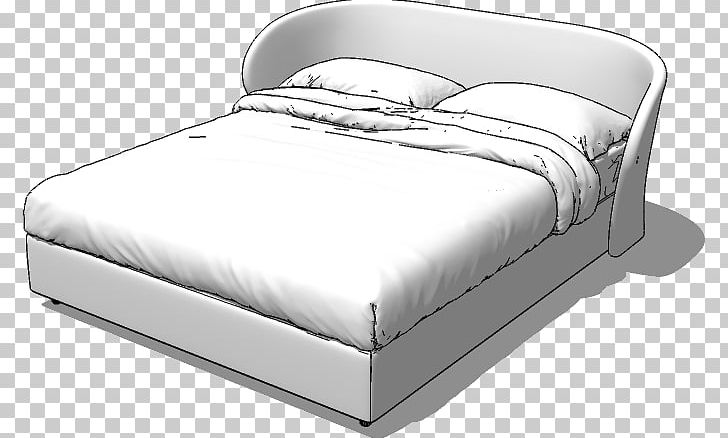The image portrays a detailed drawing of a bed set against a grey and white checkerboard background. The bed, possibly a double, queen, or king size, features a unique headboard. This headboard is thin yet gives a soft appearance as it curves around the top sides of the bed, enveloping it elegantly. Notably, the bed is depicted in a monochromatic scheme, utilizing black lines and shadowing for distinction. 

The mattress is set within a standard, square frame that matches the headboard's material, giving an impression of a consistent, soft plastic design. Covering the mattress is a thick, folded-back comforter, or duvet, revealing two pillows positioned at the head of the bed. The meticulous details continue with tight hospital corner folds at the blanket’s bottom. The overall style of the drawing is modern and minimalistic, dominated by the interplay of white, grey, and black shades, void of any text or additional embellishments.